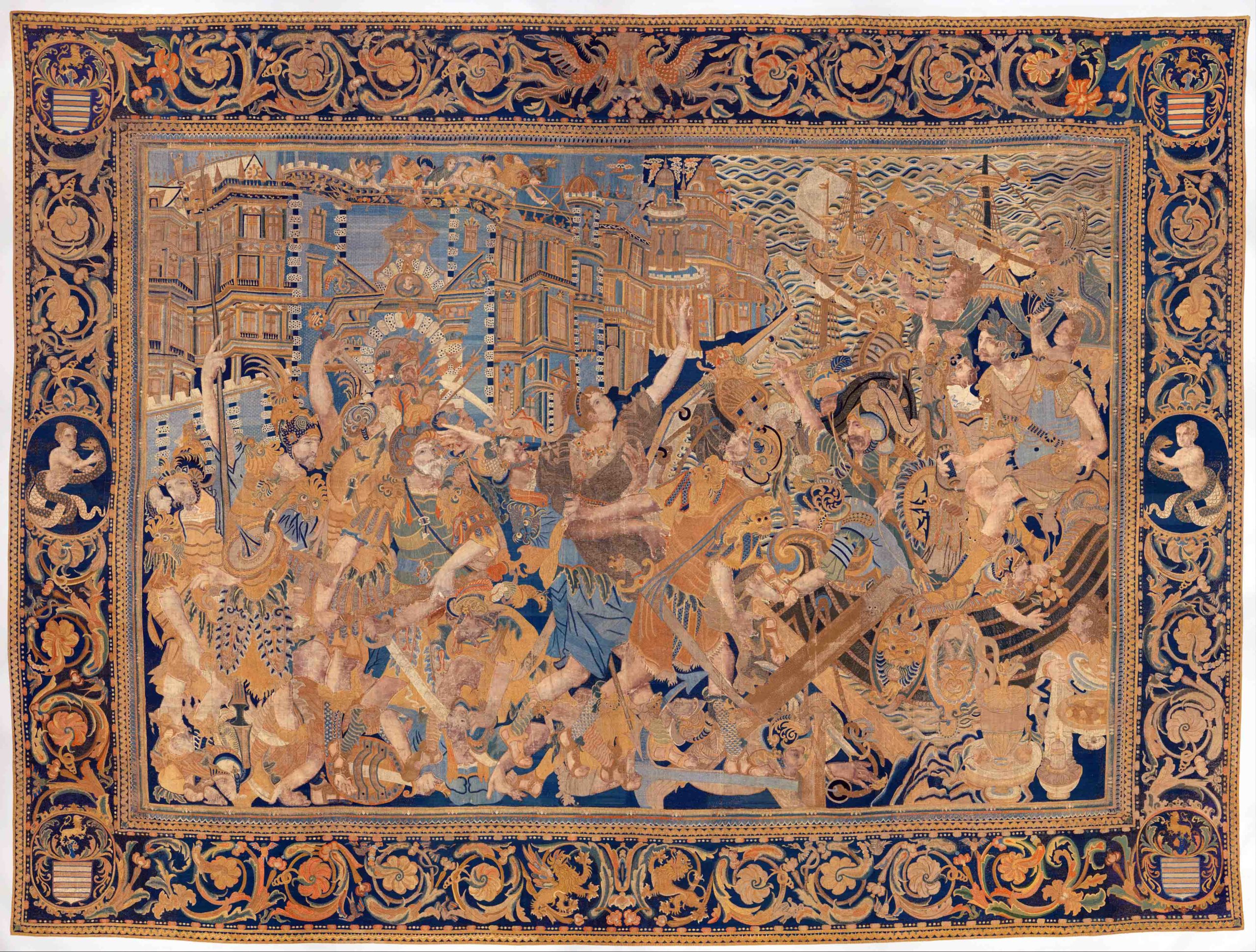This intricate and visually compelling artwork appears to be an Olden-style tapestry, richly detailed and potentially museum-quality. The tapestry showcases an ornate, thick border featuring complex scrolling ornamentation, including flowers, pillars, and cherubic figures. Unique elements such as facing lions and men holding snakes or griffins enhance the border's complexity. Each corner features a crest or emblem topped by a bird perched on a vase overflowing with shrubbery, adding to its elegance.

Within the lavish border, the central scene teems with individuals depicted in what seems to be a battle, some adorned in battle gear with primary colors of orange, navy blue, and white. The figures, some reaching skyward, others towards one another, exhibit a dynamic sense of movement. Background details include a blue castle with brown shading, atop which several figures are positioned. A portion of the upper right-hand section reveals an ocean-like expanse with a ship and a moon.

The tapestry's overall color palette includes complementary combinations of beiges, light and medium browns, with lighter and darker blues, creating an aesthetically pleasing and harmonious look. Despite the chaotic array of body parts—arms and legs intertwining—there's a cohesiveness to the imagery, punctuated by the detailed townscape in the background, following the dominant blue, brown, and gold hues. Whether viewed head-on or from above, this tapestry offers a rich, elaborate depiction that draws the viewer into its historic and artistic narrative.